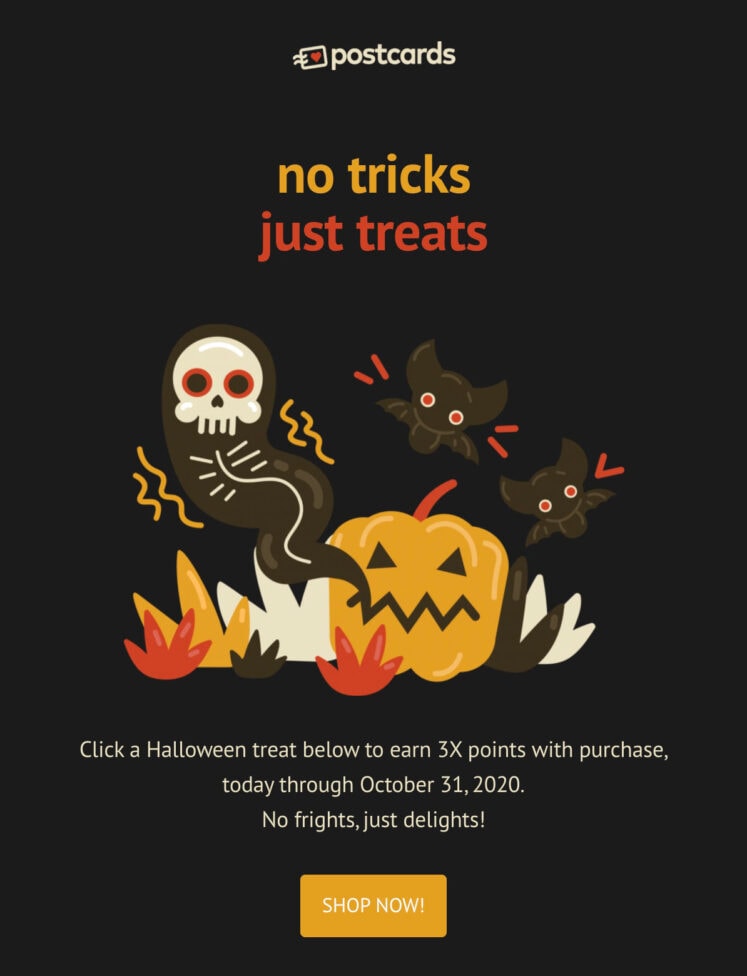Here's a detailed and cleaned-up caption for the image:

"The background of this area is solid black. At the top center, the word 'Postcards' is displayed in white text, accompanied by a small white square with a touch of red inside. Further down, in yellow text, it reads 'No Tricks,' and just below this, in red text, 'Just Treats.' The central image features an orange jack-o'-lantern with a zigzagged mouth, a red stem, and two black bats with red eyes and red-lined wings. To the side, there’s an outline of a fish skeleton with a visible long swirly line, a white skull, and red circular eyes. Along the bottom of the image are various plants colored in red, orange, black, and white. Below this visual, a message in white text encourages viewers: 'Click a Halloween treat below to earn 3x points with purchase today through October 31, 2020. No frights, just delights!' This is followed by a yellow square containing the words 'Shop Now.'"